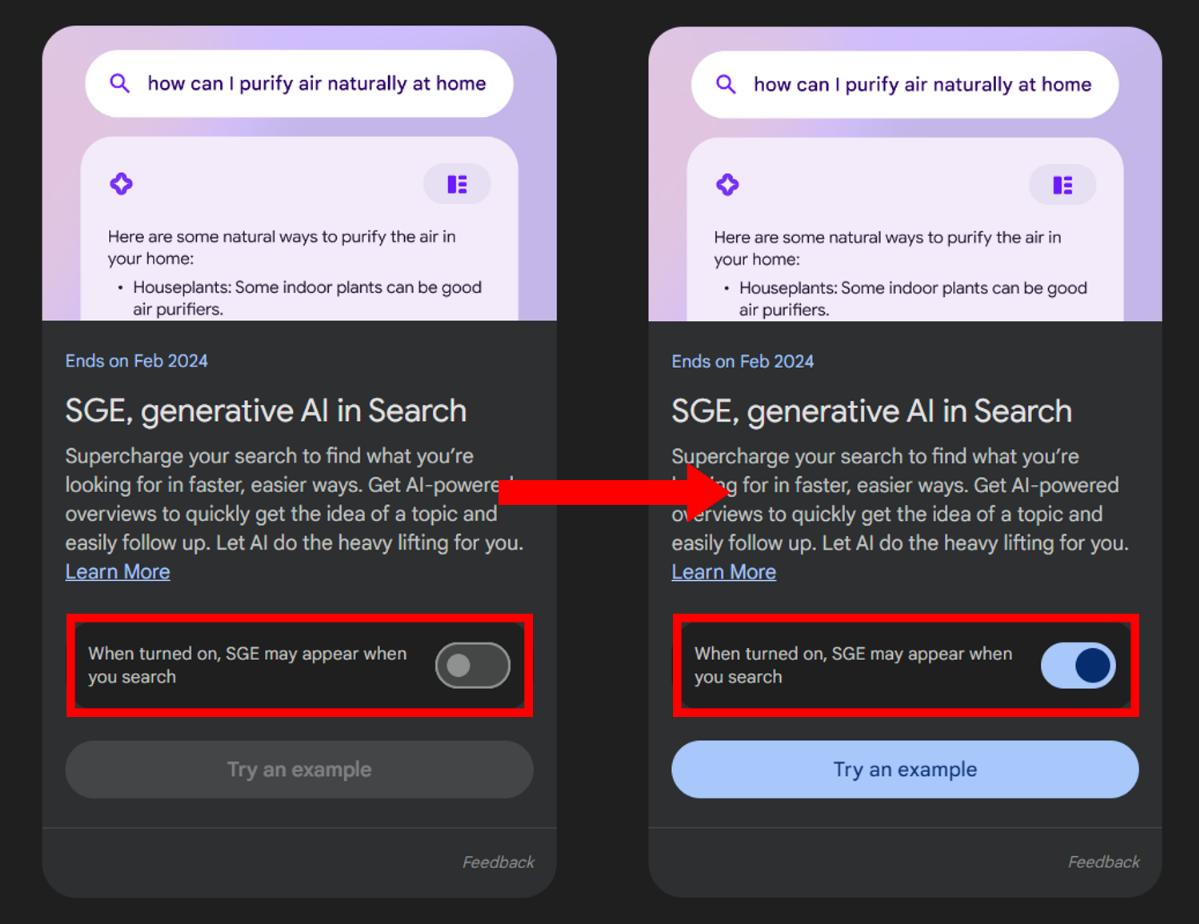The image showcases two screenshots of a mobile application with a predominantly black background. Both screenshots highlight an interface involving a generative AI feature within a search application.

The top of each screenshot features a search bar with the query, "How can I purify air naturally at home?" Immediately below, text explains various natural ways to purify indoor air, mentioning that house plants can act as effective air purifiers.

Further down the window, a promotional section introduces SGE (Search Generative Experience). It states that this AI feature can supercharge searches, helping users find information more quickly and easily. The promotion suggests that AI-powered overviews can provide quick insights into topics and facilitate easy follow-ups. A button labeled "Learn more" is included here.

In the right screenshot, the current state of SGE activation is depicted: the "When turned on, SGE may appear when you search" option is disabled (grayed out), and a "Try an example" button is also inactive (grayed out).

The left screenshot mirrors the right but shows the SGE feature activated. The previously grayed out "When turned on, SGE may appear when you search" toggle is now enabled. Subsequently, the "Try an example" button at the bottom is now highlighted in blue, indicating it can be clicked.

Both images effectively demonstrate the activation and functionality of the SGE generative AI search feature within the application.